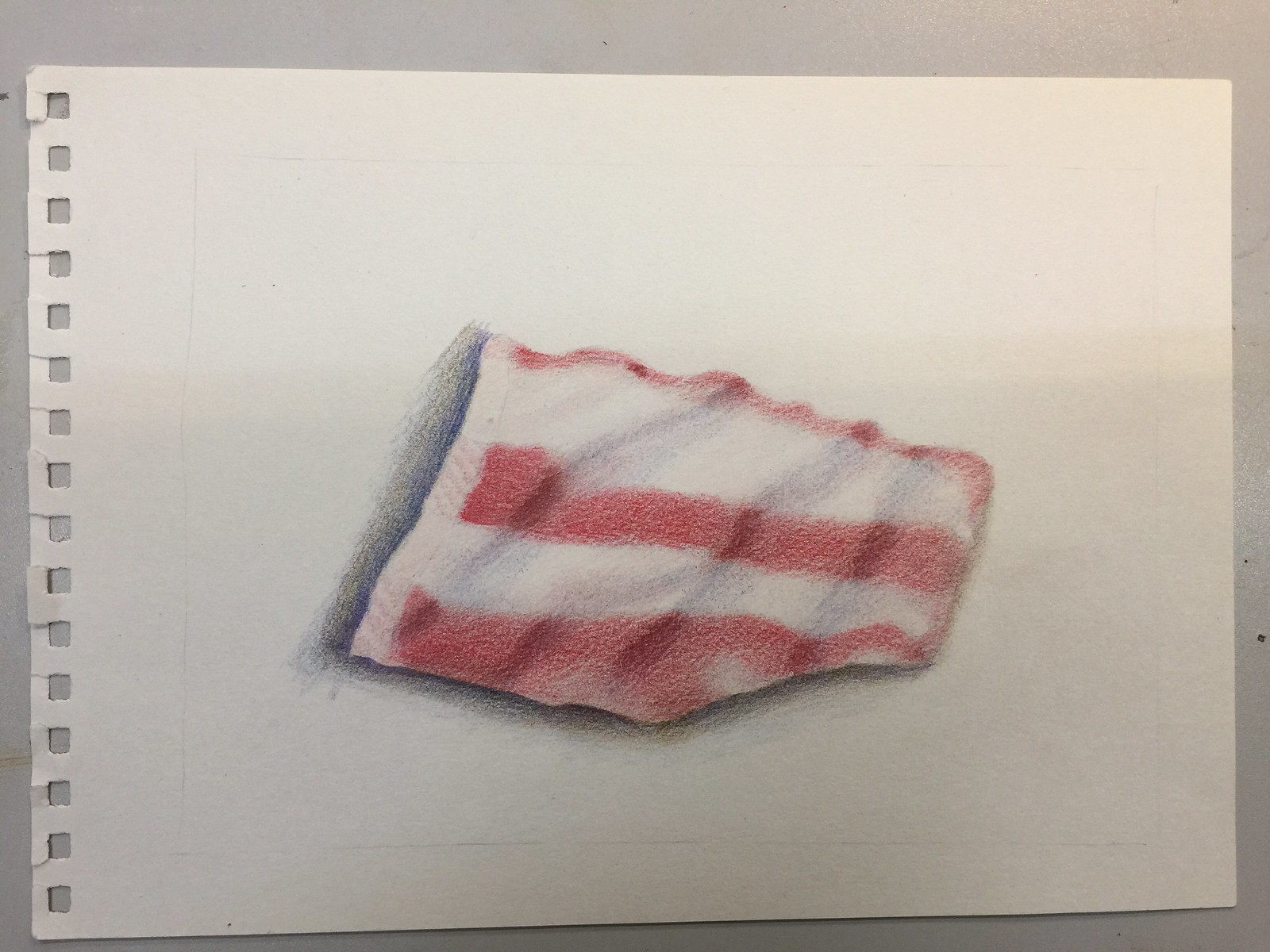In this image, there is a torn white sheet of paper that appears to have been ripped out of a spiral-bound sketch pad, as evidenced by the small, evenly spaced squares along the left edge where the paper was once attached to the rings of the pad. The edges of the paper are jagged and torn. At the center of the paper is a detailed drawing of a wavy, rectangular cloth, resembling a flag. This cloth is white in color and accented with flowing red stripes running horizontally across its surface, giving it a dynamic, rippling appearance. Shading around the sides and underneath the cloth enhances its dimensionality and suggests a sense of depth. The artwork seems to have been created using colored pencils and perhaps a graphite pencil for the shading.